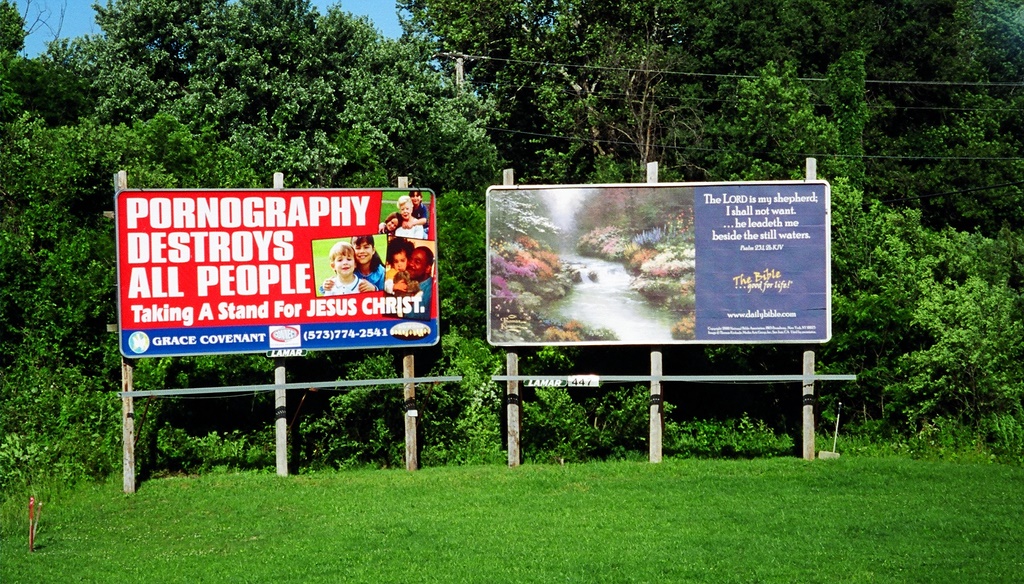This color photograph, taken during the daytime outside, features two small religious billboards erected on three wooden posts each. They are situated in a lush, green grassy area with nearby bushes and trees, with a glimpse of the sky and power lines visible in the background.

The billboard on the left has a red background with white capital letters reading, "Pornography destroys all people. Taking a stand for Jesus Christ." Below the main text is the name "Grace Covenant" within a blue border, followed by a phone number, 573-774-2541. This billboard also showcases pictures of diverse, happy families, including an older couple, a young girl and boy, an African-American man with a mixed baby, and a grandmother with two grandchildren.

On the right is a similarly sized billboard depicting a serene outdoor scene of a winding stream surrounded by colorful and lush foliage. The text on this sign quotes the Bible, stating, "The Lord is my shepherd, I shall not want. He leadeth me beside the still waters." The image features a stream meandering through rocks, with vibrant plants on either side displaying hues of purple, pink, orange, and white. The billboard includes the identifier "Lamar 447" and has additional text indicating it is from the Bible, good for life.